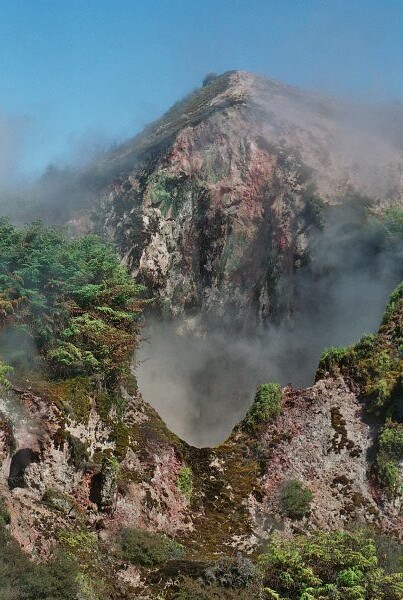The image captures a breathtaking and expansive outdoor scene set in a natural landscape, likely at a high elevation. The viewpoint is from a clifftop or mountain summit, overlooking a vast valley shrouded in dense fog or steam, possibly indicating the presence of hot springs or geysers below. In the distance, a larger, fog-enveloped mountain stands majestically against a clear, blue sky. The rocky terrain is predominantly white with reddish-pink accents, accented by green moss and a diverse range of shrubbery in shades of green, white, red, and beige. There are no animals or humans present, allowing the pristine, tranquil beauty of the natural environment to shine through. The scene is vividly rendered in an array of natural colors, including greens, browns, reds, grays, and blacks, offering a detailed and stunning landscape view of a mountainous region.